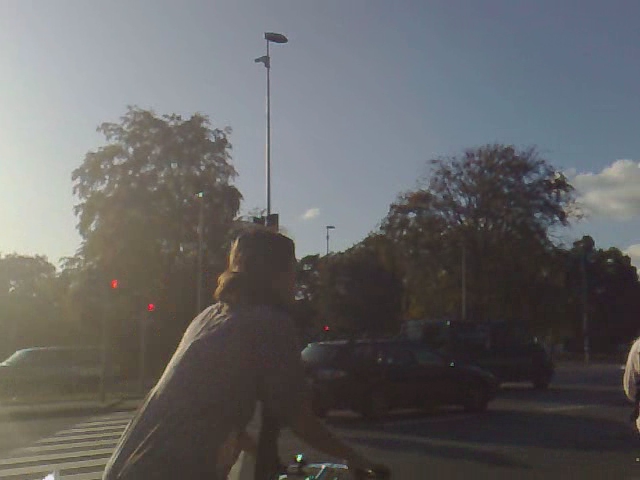This photograph has a nostalgic, faded aesthetic reminiscent of vintage photography. It depicts a white woman with brown hair tied in a low ponytail or bun, riding a bike on a busy street. The woman, dressed in a light purplish dress and scarf, is situated slightly to the left of the center, visible from the waist up, with the bike’s handlebars just in frame. 

Behind her, to the left, is a crosswalk and a set of traffic lights glowing red. A car is driving off towards the left side of the image, while two other vehicles, a station wagon and a boxy van, move towards the right. The background features lush green trees under a blue sky dotted with a few clouds. A street lamp seemingly emerges from behind the woman's head, though it remains unlit due to the daytime setting. On the far right edge of the frame, the arm of an unidentifiable pedestrian is just barely visible, adding an element of everyday life to the scene. The location of the photograph remains ambiguous.